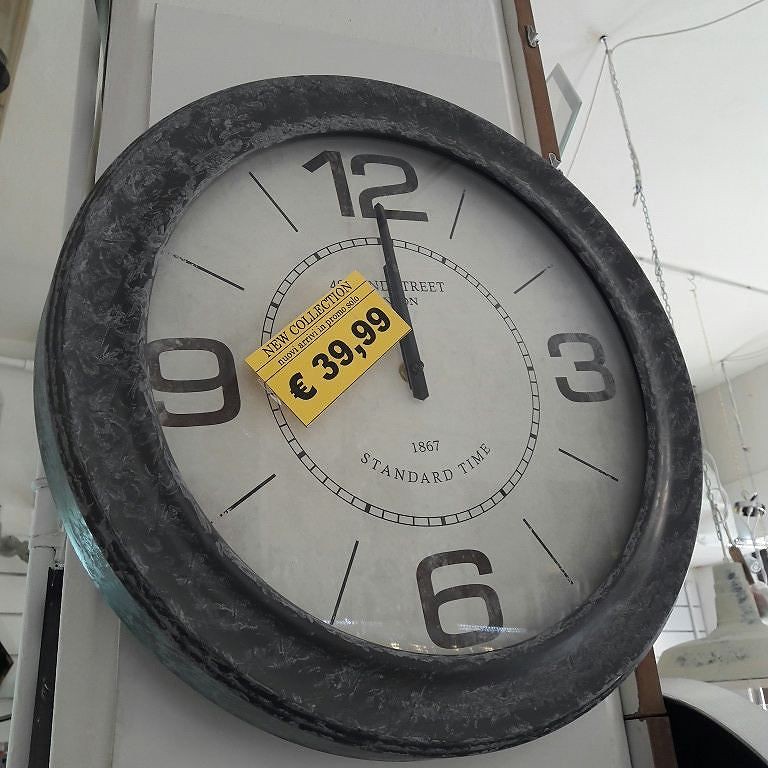The image features a prominently displayed clock, seemingly designed to resemble an antique, affixed to what looks like a support beam or white wall within a store. The beam stands in contrast to the white ceiling, which features silver chains hanging down, likely connected to light fixtures. To the left, a white pole can be seen descending, while the right side shows some protruding wooden boards.

The clock is round with a weathered, dark grey circumference that mimics the look of black granite, complete with swirls of grey that add to its rustic charm. The clock face is white and centrally positioned, bearing black numerals, specifically the 12, 3, 6, and 9, with lines indicating the other hours. Below the center, it reads "1867 Standard Time." A notable addition is a yellow rectangular price sticker near the 9, which states "New Collection" and lists the price as €39.99. Some Italian text is visible below the promotional phrase, emphasizing its new arrival in the collection. Overall, the focal point of this image is the aged-looking clock, set against a clean, white background, creating a stark yet intriguing visual contrast.